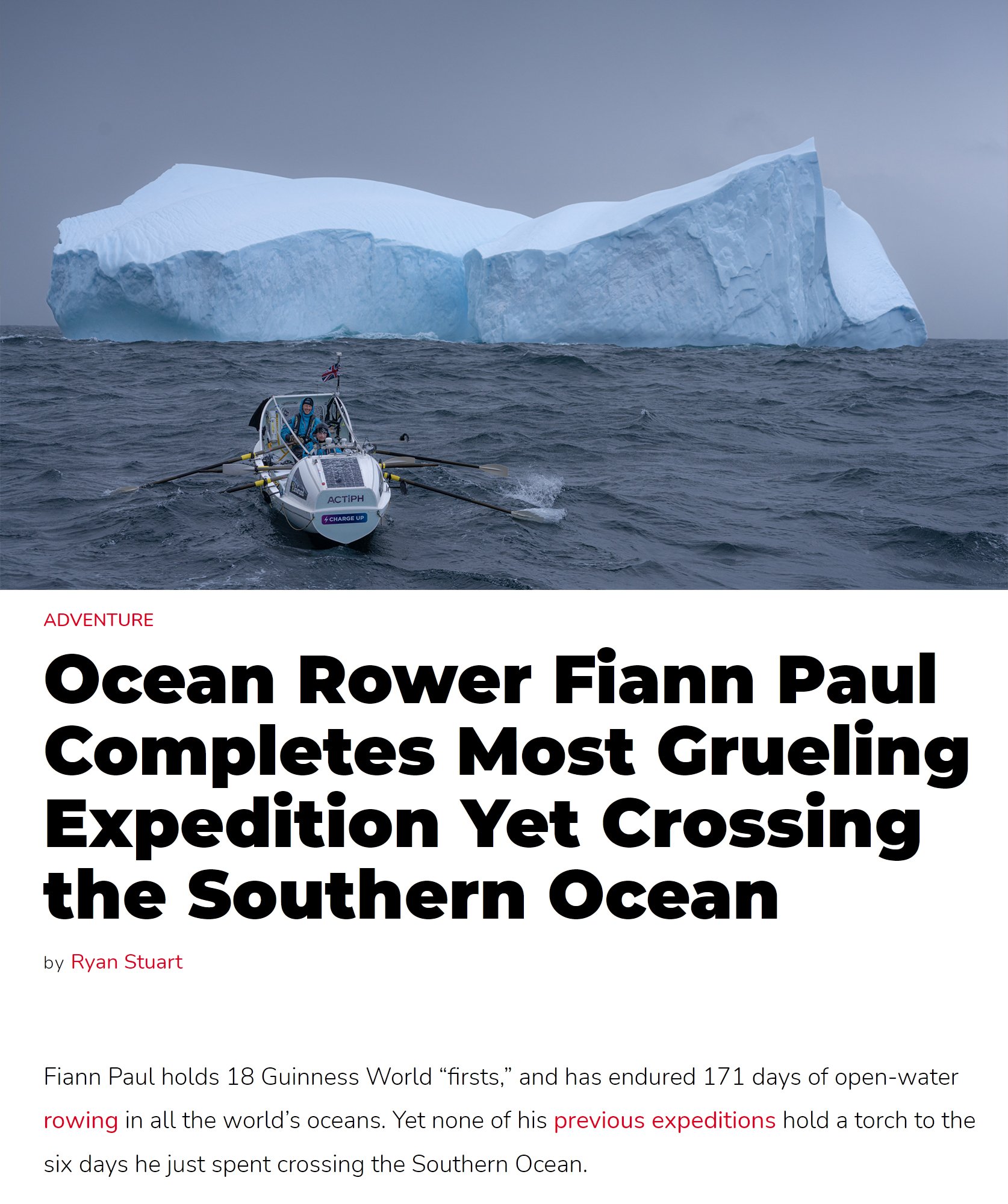The image is a screenshot of a news story featuring a striking photograph and detailed text. At the top of the image, a photo captures a small rowboat with two people in blue jackets, navigating choppy blue waters toward a colossal, floating iceberg under an overcast gray-blue sky. The scene conveys the vastness and peril of the ocean expedition.

Below the image, the headline, in black and red text, reads: "Ocean Rower Fionn Paul Completes Most Grueling Expedition Yet, Crossing the Southern Ocean." It is noted that Fionn Paul holds 18 Guinness World Records and has endured 171 days of open-water rowing across all the world's oceans. However, none of his prior expeditions compare to the six harrowing days he recently spent crossing the Southern Ocean. The article is credited to Ryan Stewart, whose name appears in red text.